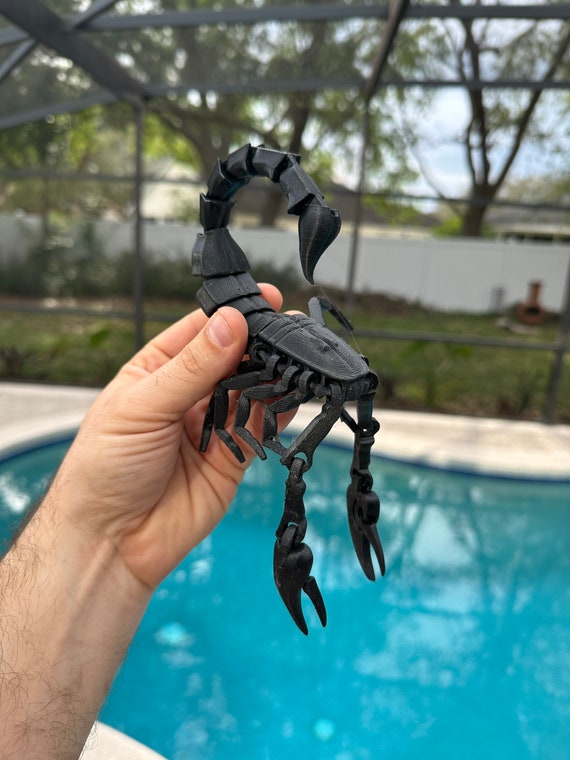In this detailed image, a man's hairy arm extends from the left side, prominently displaying a lifelike, black metal scorpion. The scorpion, boasting intricate details such as a curled tail, prominent claws, and downward-hanging legs, appears poised for action with its stinger raised in a striking pose. Behind this striking object, the serene setting of a backyard pool is visible. The water is a vibrant blue, accentuated by surrounding marble tiles. Further in the background, the scenery unfolds with a fence enclosing a lush area full of trees, lending a picturesque and tranquil atmosphere to the scene.